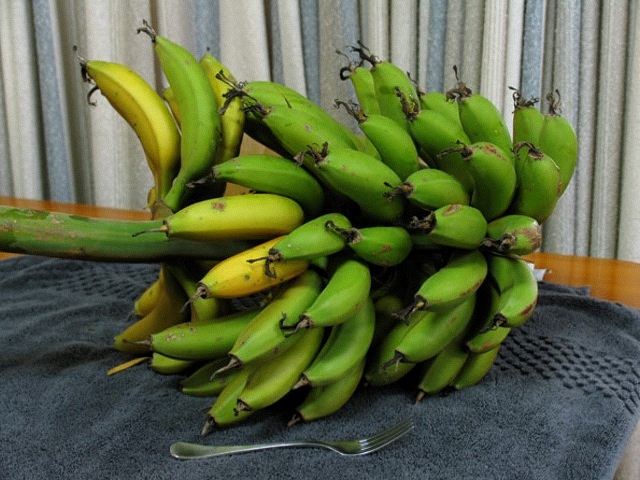In this photo, a large bunch of bananas, still attached to the tree limb, is displayed on a wooden tabletop covered with a blue blanket adorned with diamond-shaped studded designs. The bananas are predominantly green, indicating they are far from ripe, with a few yellow bananas visible at the bottom and to the left, suggesting they are starting to ripen. In the foreground, a silver or stainless steel fork lies in front of the bananas. The background features a combination of white, blue, and gray curtains. The setup captures the bananas with the bottom parts facing the camera and the tops pointing away, adding depth to the composition.